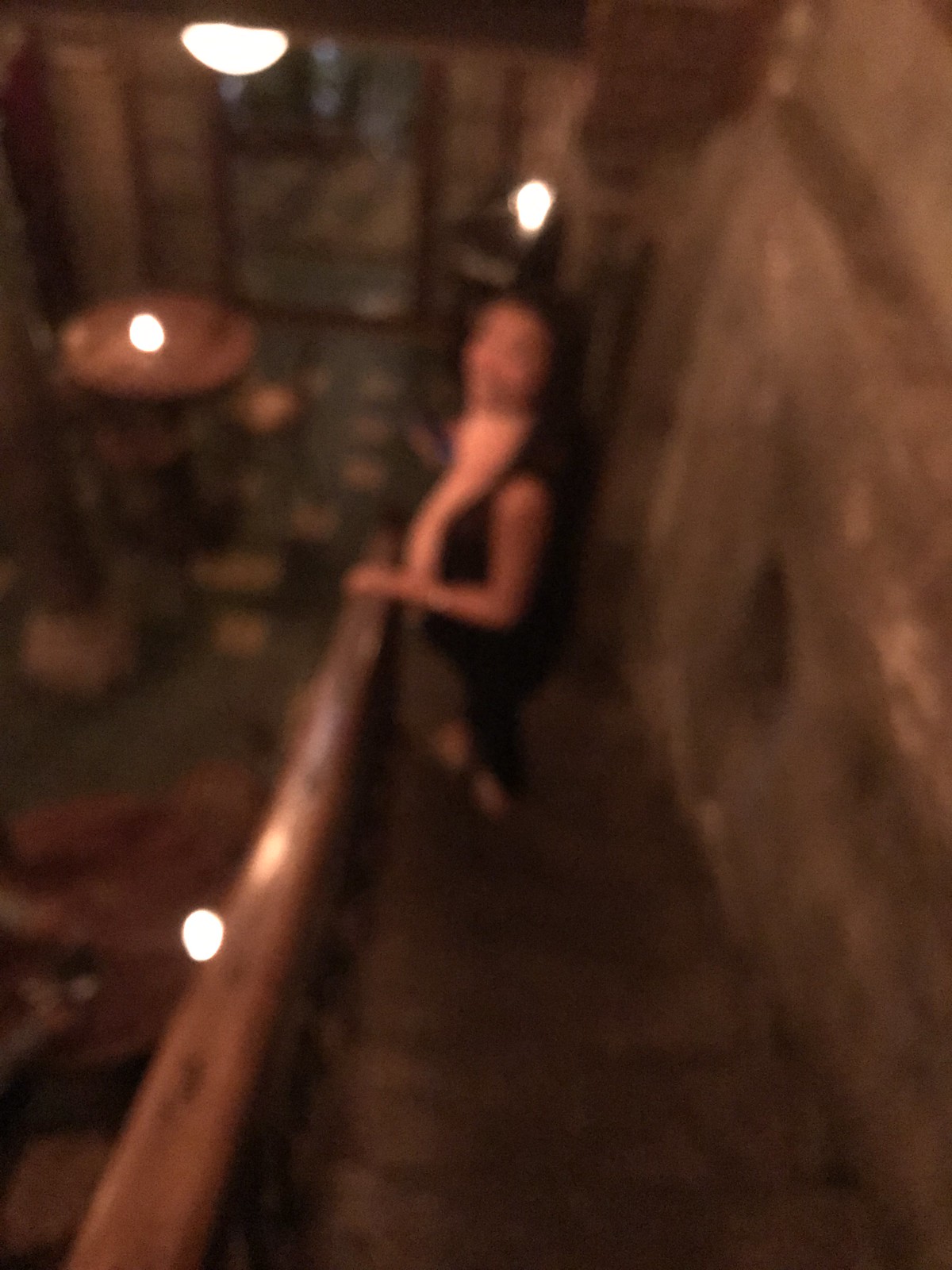In the extremely blurry photograph taken in a dimly lit room, the main focus is a staircase with brown steps and a lighter brown railing. The camera is positioned above, looking down towards the bottom of the stairs. To the right of the image, there is a wall in a grayish brown or brownish gray hue, with patches of white. At the bottom of the stairs, a woman, dressed in a black jacket, white shirt, and black pants, stands looking up at the camera. Despite the blur, her smiling face is vaguely discernible. She has dark hair and is possibly holding onto the railing with her left hand. The scene includes a circular wooden tabletop to the left of the image and a door that presumably leads outside behind the table. The area is dimly lit, possibly by ceiling lights or a candle on the table.